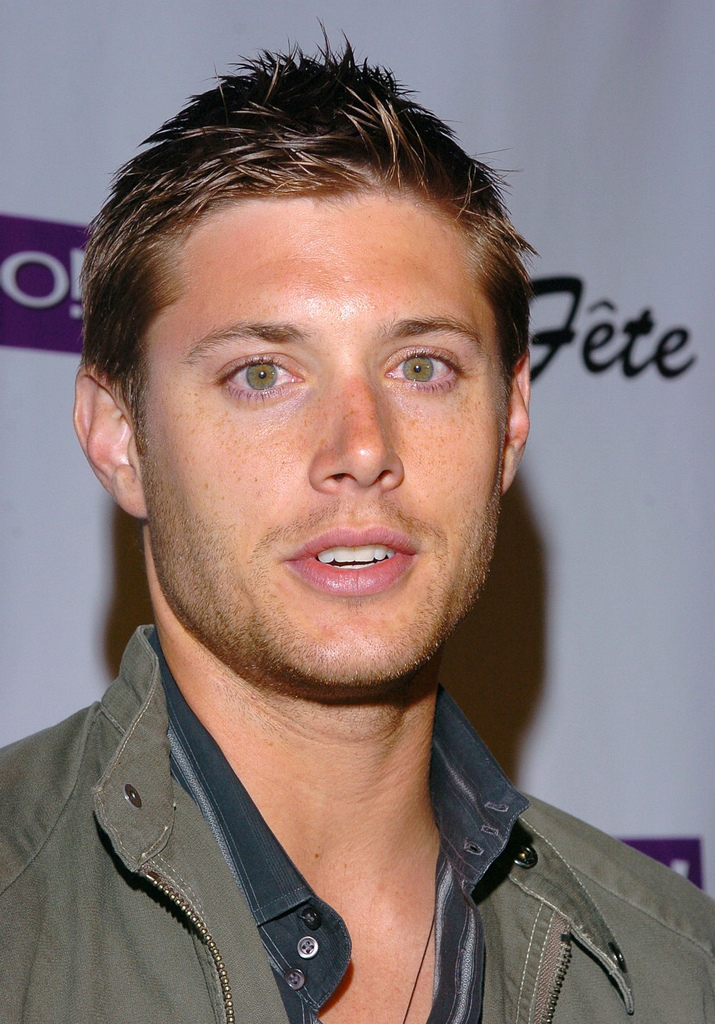This is a close-up headshot of a young Caucasian man in his early 20s, likely one of the actors from the show "Supernatural." He has fair skin with a slight stubble beard, a light mustache, and his mouth is slightly parted as if he might be about to speak or smile. His hair is blondish-brown, short, and spiked slightly at the front while cut closely on the sides. His striking blue-green eyes stand out, giving him a very handsome appearance. He is dressed in a green jacket with a zipper and buttons around the collar, over a blue collared shirt with a few buttons undone, revealing a thin silver chain necklace that dips below the frame. The background features a white promotional wall typical of red carpet events, adorned with a purple Yahoo logo or possibly black lettering that spell out "F.E.T.E." The bright flash from the camera casts a shadow behind him on the wall, highlighting his well-groomed features.